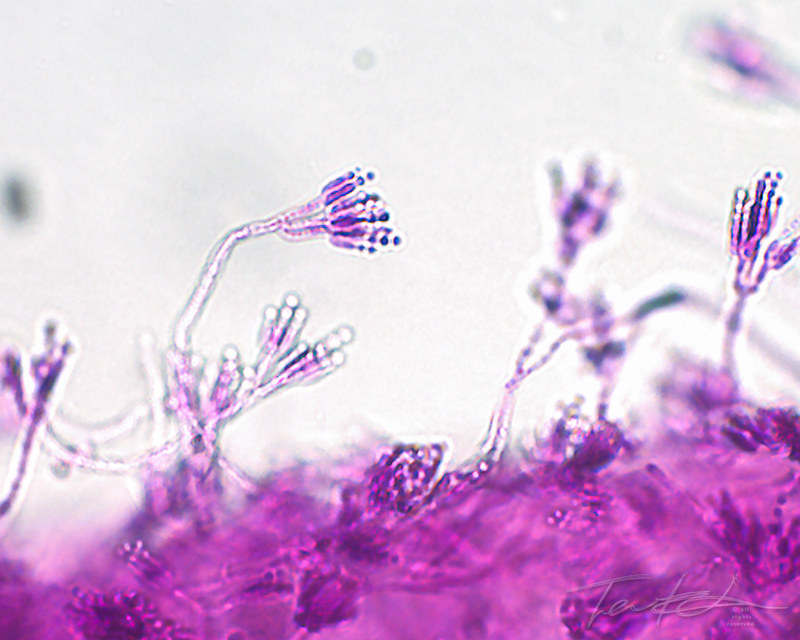The image appears to be a highly detailed, vibrant purple, microscopic view of cellular material resembling flowers. These cellular structures have stem-like bases with circular, floral shapes at their ends, which are predominantly clear-colored. The dominant, chaotic textures and bright, elegant hues of purple contrast against a white background, adding to the image's striking visual complexity. Notably, the resolution becomes pixelated and noisy in regions with the floral shapes. A cursive signature, possibly the author's, is present in the bottom-right corner, along with a watermark.